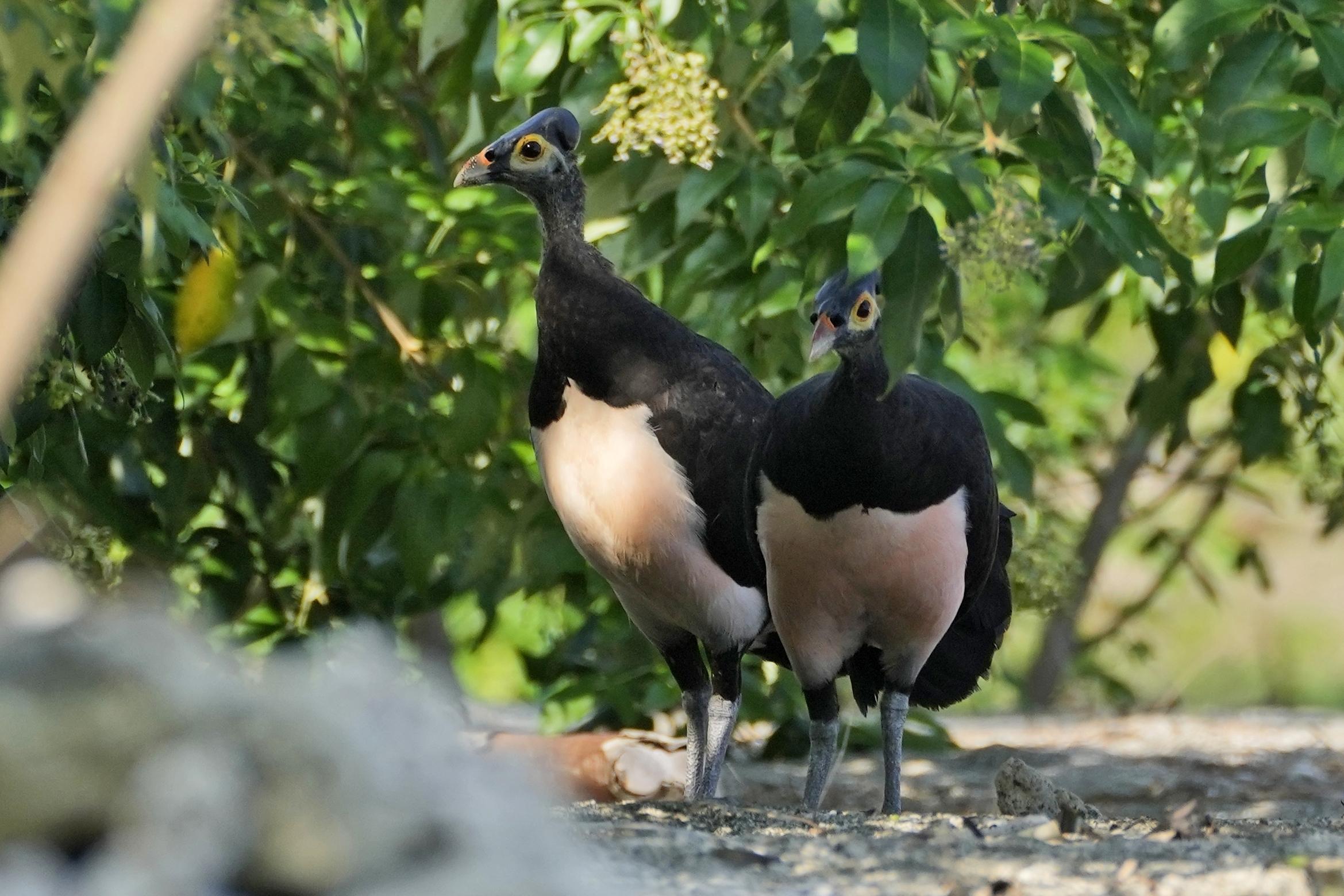This photograph captures two distinctive, large birds standing side-by-side on a gravel-like ground, possibly outdoors. Each bird, primarily black with an off-white chest, exhibits unique and intricate details. Their black heads are adorned with small mohawks, accented by a semi-circular orange pattern over the eyes and around their short, pointed beaks which also feature an orange stripe. The area around the birds’ eyes is a lighter shade of gray and the eyes themselves are a dark brown. They stand on twig-like legs, grayish in tone, that transition to black at the top. The setting appears serene, with sunlight filtering through trees and bushes, casting shadows around the birds, emphasizing their curious stance. Leaves from the plants enhance the natural background, providing a contrast to the stony ground they are on. Despite being outdoors and seemingly away from urban scenery, the organized terrain and surrounding flora hint that this could be within a managed environment, possibly a zoo.